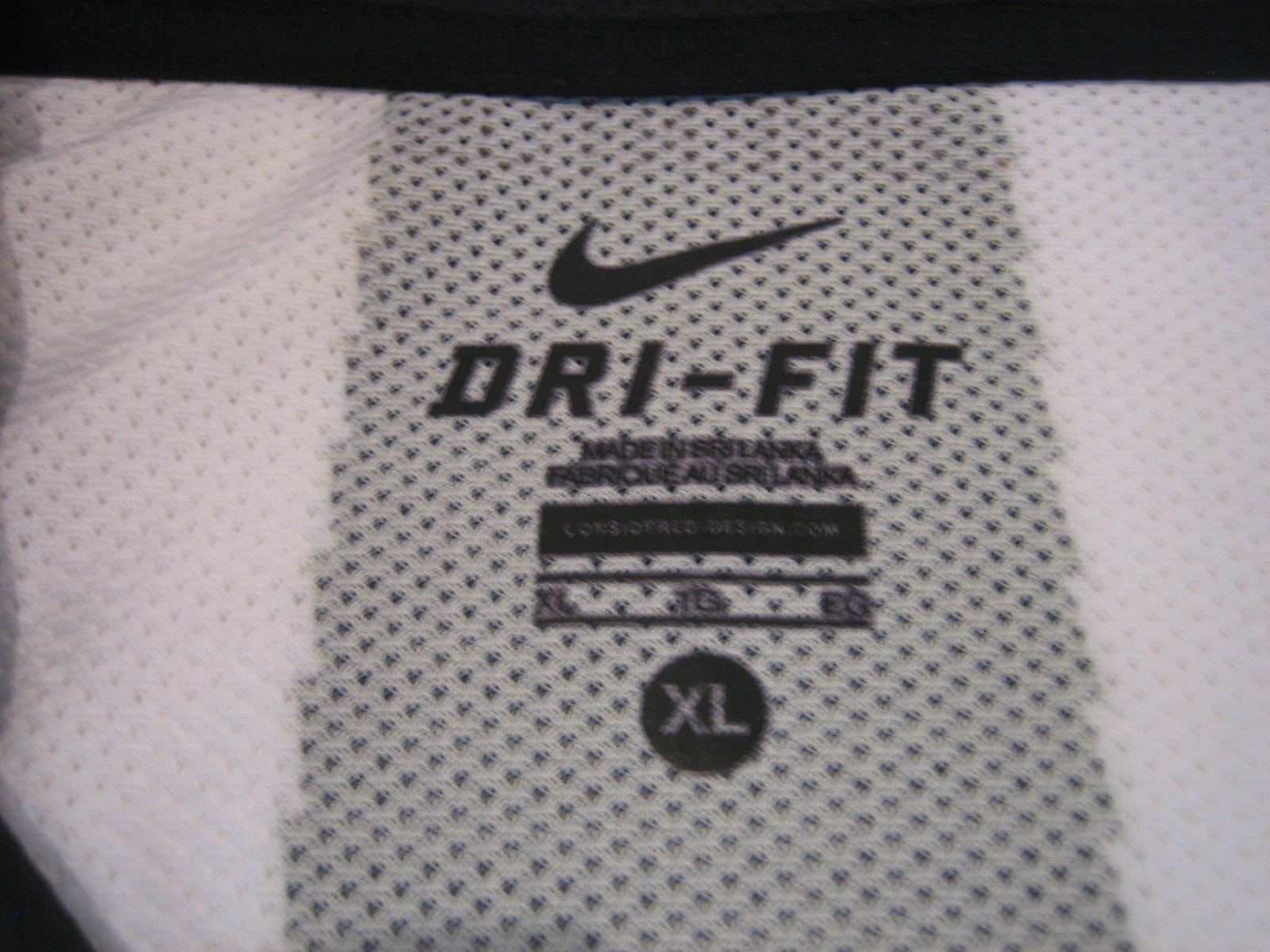This is a detailed photograph of a high-quality athletic garment. The garment features three panels: the outer panels are white, while the central panel is gray. Positioned at the top of the garment is a black check mark, suggesting it might be a Nike item. Below the check mark, the word "Dri-FIT" is printed in black font, denoting the fabric technology. Further down, it states "Made in Sri Lanka" in black font, although this text is slightly blurred. The size information, "XL," is displayed in a black circle with lighter-colored font. Each panel of the garment is adorned with small mesh circles, showcasing the breathability and softness of the fabric. Despite a minor blur over the "Made in Sri Lanka" text, the overall image quality allows for the discernment of individual mesh circles, highlighting the garment's excellent craftsmanship.